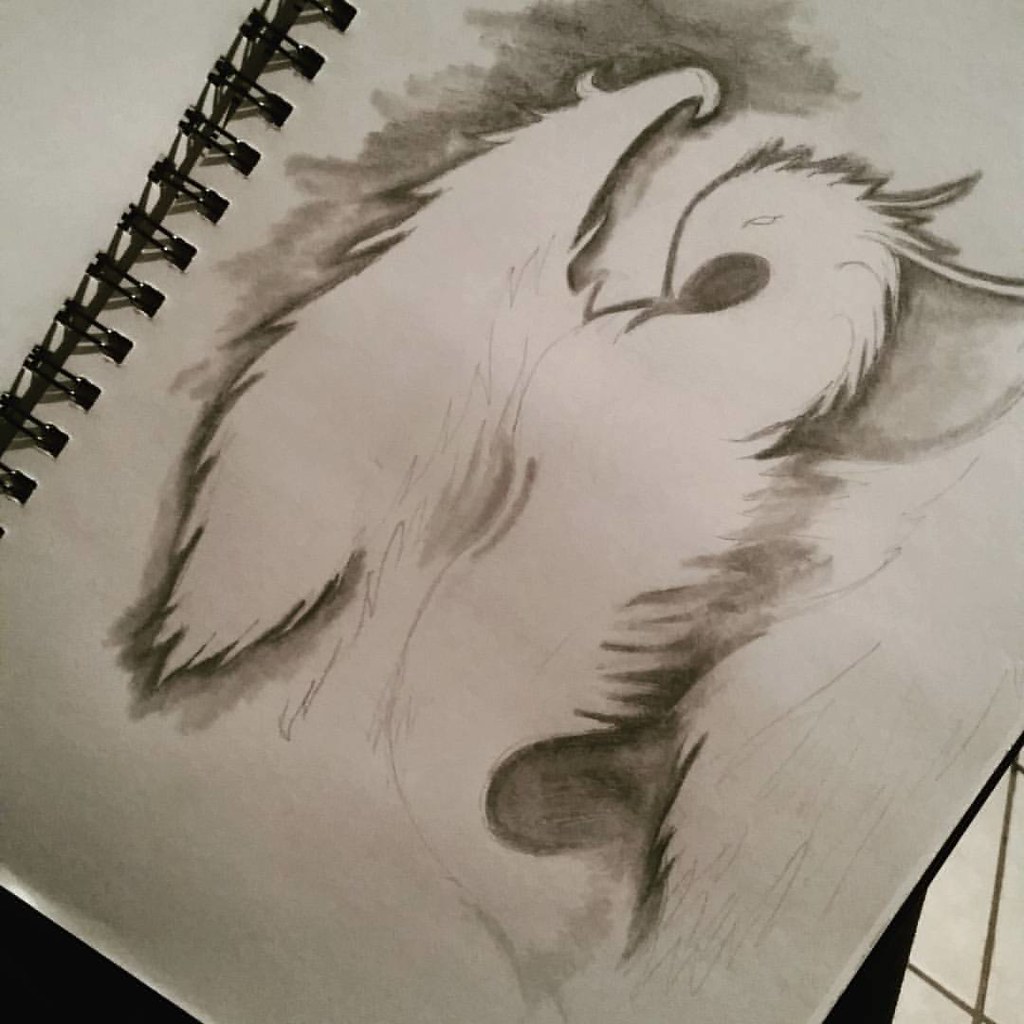A detailed depiction of a sketchbook with spiral binding on one side, captured at an angle that places it in a diagonal orientation. The page reveals a delicate drawing, potentially of a phoenix or dragon, characterized by its notable outline and subtle feathering. The creature features expansive wings, a sinuous body, and an elegantly arching neck that terminates in a sharp beak. The head includes a small eye, and the edges of the figure exhibit a shaggy texture, suggestive of feathers. Though the drawing lacks intricate details, it boasts exquisite shading behind the wings, body, and head, imparting a sense of depth and grace to the mythical being.